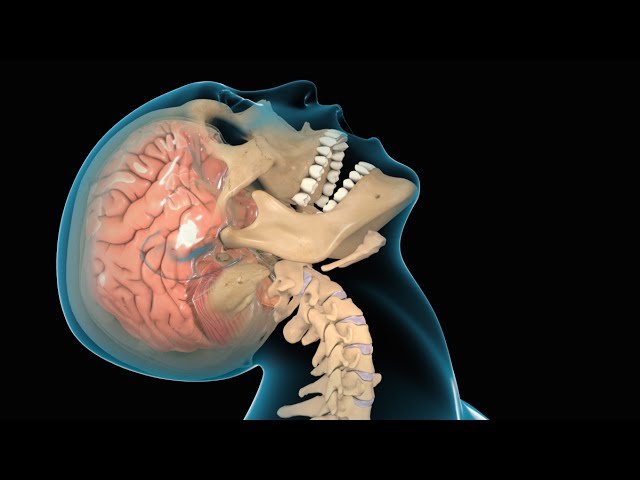The image is a highly detailed medical depiction featuring the translucent, bluish-black silhouette of a human figure centered against a completely black background. The subject's head is tilted back, eyes closed, and mouth open, conveying an expression as if looking towards the sky or ceiling. Within this translucent form, the intricate anatomy of the person is revealed: a pink brain with blue-tinted areas and visible arteries or veins, emphasizing a network of dull blue lines. The skull and teeth are stark white, contrasting against the ethereal outline. The neck is arched back, highlighting the spine's vertebrae in a plastic beige color. The muscles also stand out within the translucent form, adding depth to the anatomical model, which is not an actual person but a detailed representation. The image provides a clear side profile, displaying the head, brain, and part of the neck's vertebrae, with a notable hole where the right eye would be, offering a comprehensive inside view of the skull's bone structure and internal components.